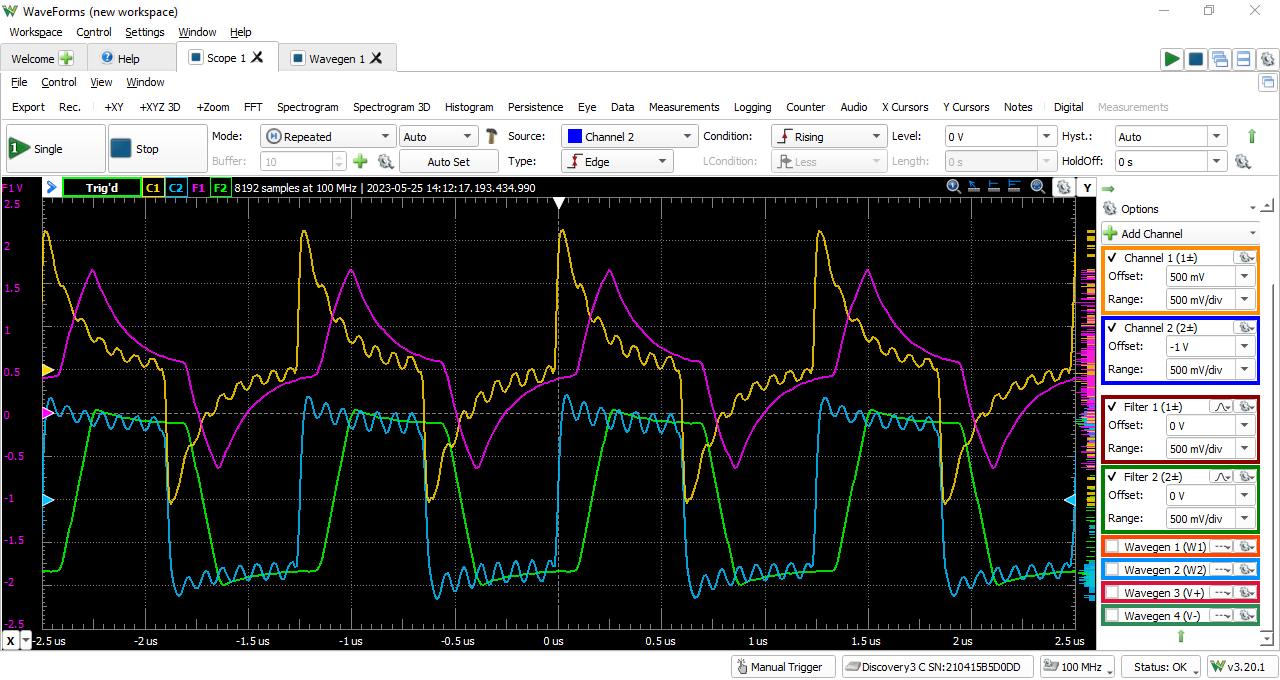This image is a detailed screenshot of a waveform analysis program on a computer, likely showcasing data from an oscilloscope. At the top of the interface, the menu bar includes tabs labeled Waveforms, New Workspace, Control Settings, Window, and Help. Below this, there are several sections named Welcome, Help, Scope 1, and Wave Gen 1, followed by an extensive list of functionalities such as File, Control, View, Window, Export, Record, X, Y, Z, 3D, Zoom, FFT, Spectrogram, Spectrogram 3D, Hologram, Persistence, Eye, Data, Measurements, Login, Counter, Audio, X cursors, Y cursors, Notes, Digital, and Measurements. 

On the right side, the interface features various drop-down tabs containing adjustable parameters and settings, highlighted by orange, blue, red, and green borders for easier differentiation. Prominent elements include offset ranges displayed in black text on a white background, a set of dials, a play button marked "Single," and a stop button labeled "Stop."

Centrally, the screen presents a black background grid displaying multiple waveform lines in different colors: green, blue, purple, and yellow. Each line represents a distinct channel with the green line appearing more stable, the blue line jagged, and other colors indicating varied waveform behaviors. This intricate graph illustrates data patterns over time, essential for analyzing signals in scientific experiments or technical diagnostics.